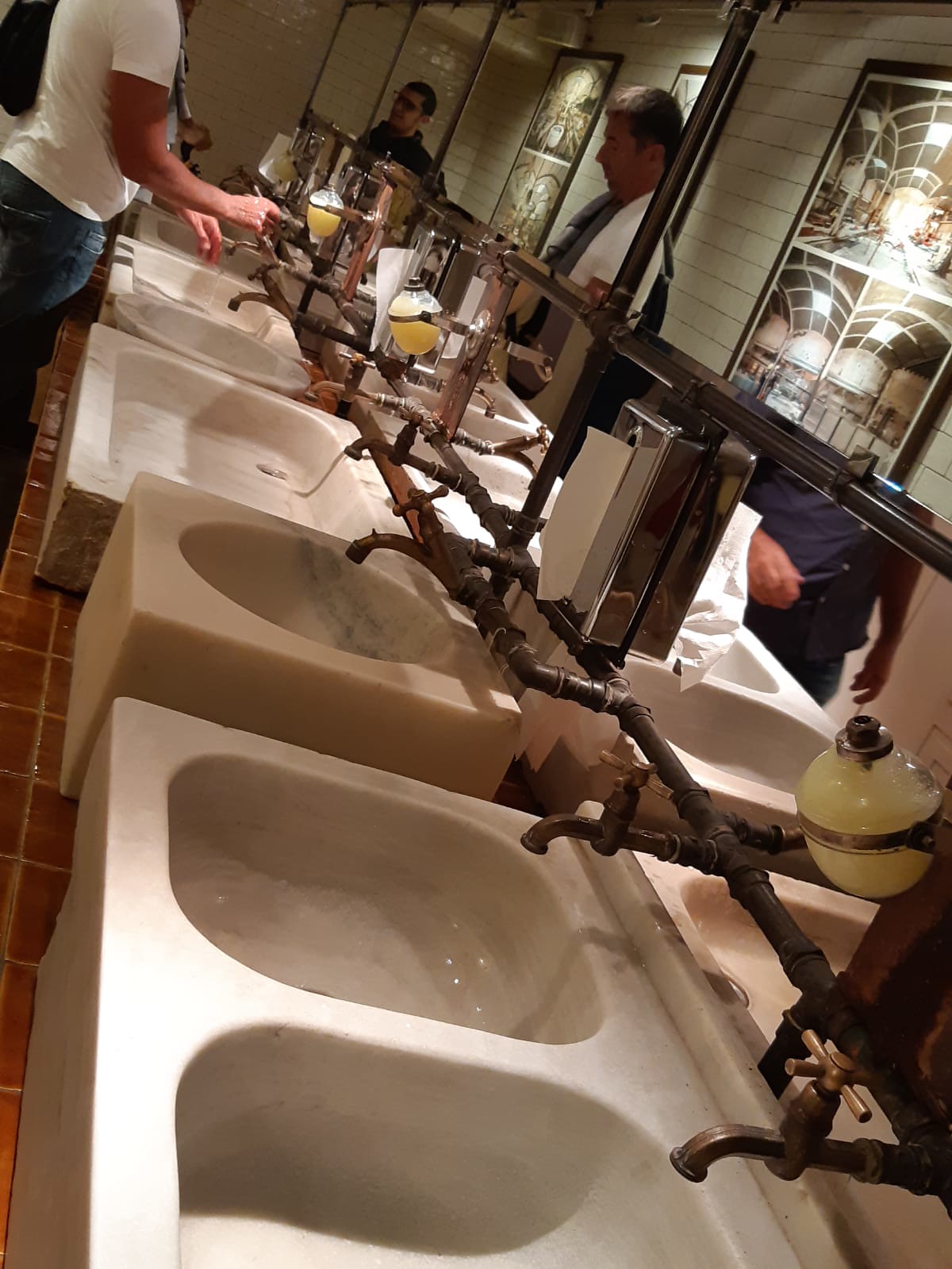This image captures an unusually designed bathroom with a nostalgic 1940s flair. The bathroom features a long row of mismatched sinks, including one resembling a twin sink, a toilet bowl, a bathtub, and a sphere, each creatively connected by a complex brass piping system. The setup creates an illusion of reflections due to the back-to-back rows of sinks, but it’s actually a large bathroom with a mirrored layout. The walls are adorned with white bricks, accented by small stained glass windows, and supporting a collection of framed photographs or paintings. The flooring is a striking red tile that complements the marble sinks. Various soap dispensers and jars filled with soap dots the area, with soap dispensers uniquely shaped like orbs or grenades. There are also tissue boxes and hand-drying stations scattered throughout. In this scene, two men are preparing to wash their hands – one in a white t-shirt and blue jeans, and another in a long-sleeved white shirt and tie, adding a human element to this intriguing bathroom setup.